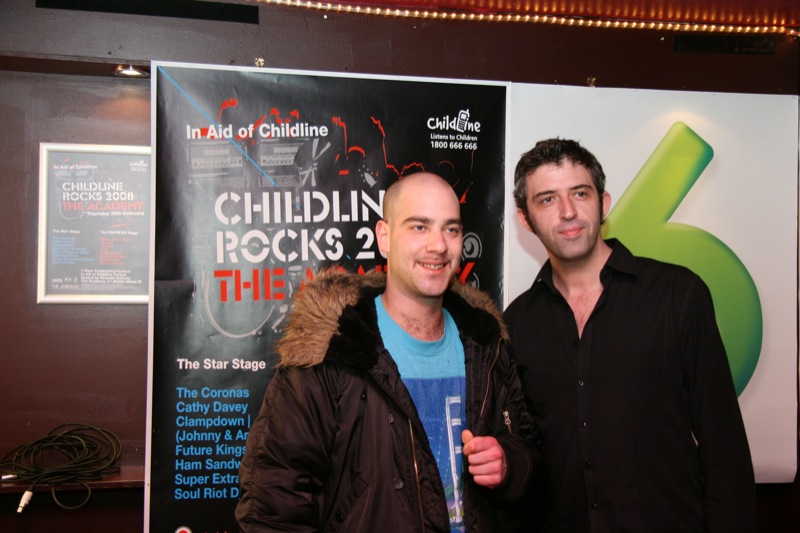The photograph, taken in the lobby of a theater, depicts two men standing together, possibly attending a benefit event for Childline titled "Childline Rocks 2008," held at a venue likely called the Aladdin. It appears to be wintertime, as suggested by their attire. The man on the left, smiling and giving a thumbs-up, is bald with close-cropped hair. He is wearing a brown parka with a tan fur collar over a blue t-shirt with a light blue top and darker blue bottom. The man to his right, with a five o'clock shadow and short dark hair graying at the sides, wears an unbuttoned black collared shirt with long sleeves. Both are looking off to their left (our right). Behind them is a black poster featuring white, red, and blue text. It mentions "in aid of Childline" with a phone number 1-800-666-666. The event they're attending, "Childline Rocks 2008," is advertised, showing several musical acts such as The Coronas, Kathy Davey, Clampdown, Johnny (partially obscured), Future Kings, Ham Sandwich, Super Extra, and Soul Riot. The larger poster's date is blocked by the bald man's head, but a smaller adjacent poster confirms the year as 2008 and location name as "The Aladdin." The scene captures a moment of community spirit and support for Childline's cause.